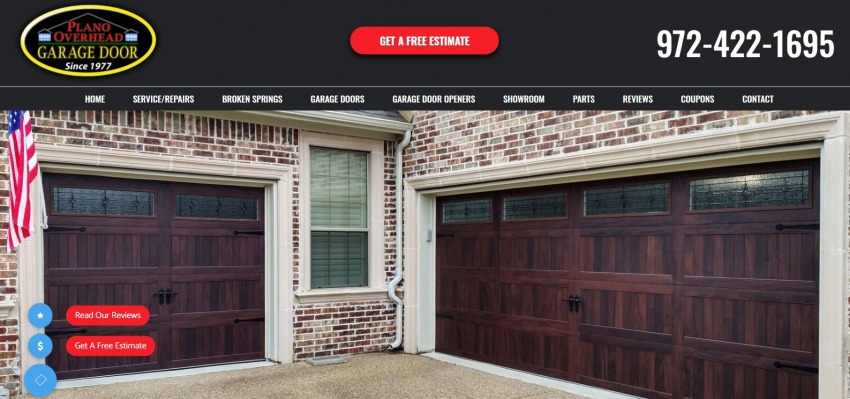The image appears to be a screenshot of a website's landing page for Plano Overhead Garage Door. The header section of the page features a very dark gray or black rectangle with an oval logo centered at the top. The logo has a shiny, yellow-gold border and a black interior. Inside, "Plano Overhead" is written in red font, "Garage Door" in yellow-gold font matching the border, and "Since 1977" in white font.

Beneath the logo, a prominent red, capsule-shaped button reads "Get a FREE Estimate" in white font. To the right, the phone number "972-422-1695" is displayed in large, bold white font. The menu bar below this includes options for Home, Service Repairs, Broken Springs, Garage Doors, Garage Door Opener, Showroom, Parts, Reviews, Coupons, and Contact.

Below the header is an image of two garage doors on a brick house. The garage doors appear to be dark wood panels with a slight reddish-pinkish-purple sheen. The brick on the house exterior is a mix of red, gray, and tan with white mortar. An American flag hangs on the left side of the house near the smaller one-car garage door. Adjacent to it is a larger, multi-car garage door, approximately twice the width of the smaller one.

Further down the page, there are two additional red, capsule-shaped buttons with white text that say "Read Our Reviews" and "Get a FREE Estimate." The section also features blue circular icons; one contains a star, another a dollar sign, and the third a square.